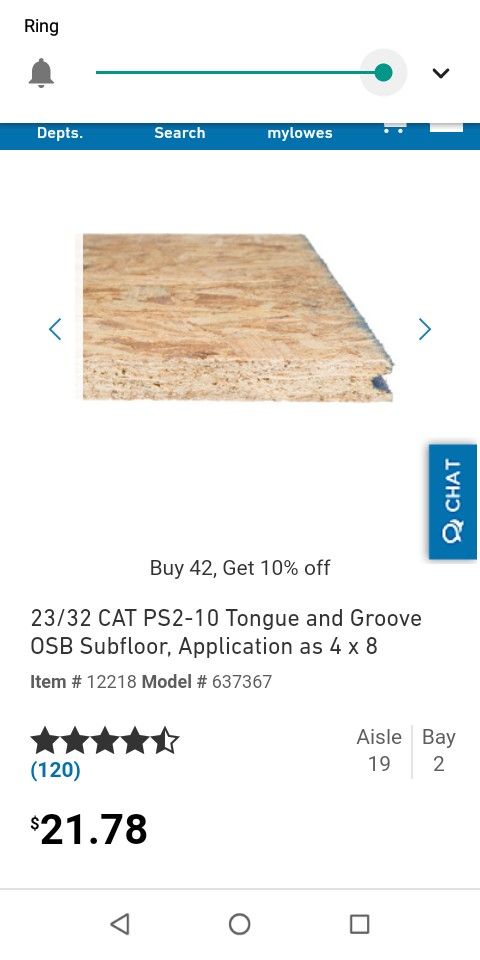Image Caption:
This image showcases a detailed view of a subfloor product and its purchasing options. At the top, there is a ring icon followed by a bell icon. Adjacent to these, a green bar features a movable circle slider positioned at the far right. Below this bar, a clickable dropdown arrow is located on the right side.

Further down, on a blue background, the text reads "Departments," and next to it is a search bar labeled "Milo's." Beneath this, there is an image of the subfloor product displayed on a white background. The subfloor is depicted as a square piece of wood with blue directional arrows pointing left and right.

To the right side of the image, there is a vertical blue chat button with the word "Chat" written vertically. Below this button, there is a horizontal banner that reads, "Buy 42, get 10% off."

The product is described in detail: "23/32 CAT PS 210 Tongue and Groove OSB Subfloor, 4x8." The item number is 12218, and the model number is 637367. The product boasts an impressive rating of 4.5 stars based on 120 reviews, with the note "Aisle 19, Bay 2" located to the right in parentheses. Finally, the price of the subfloor is prominently listed at $21.78.